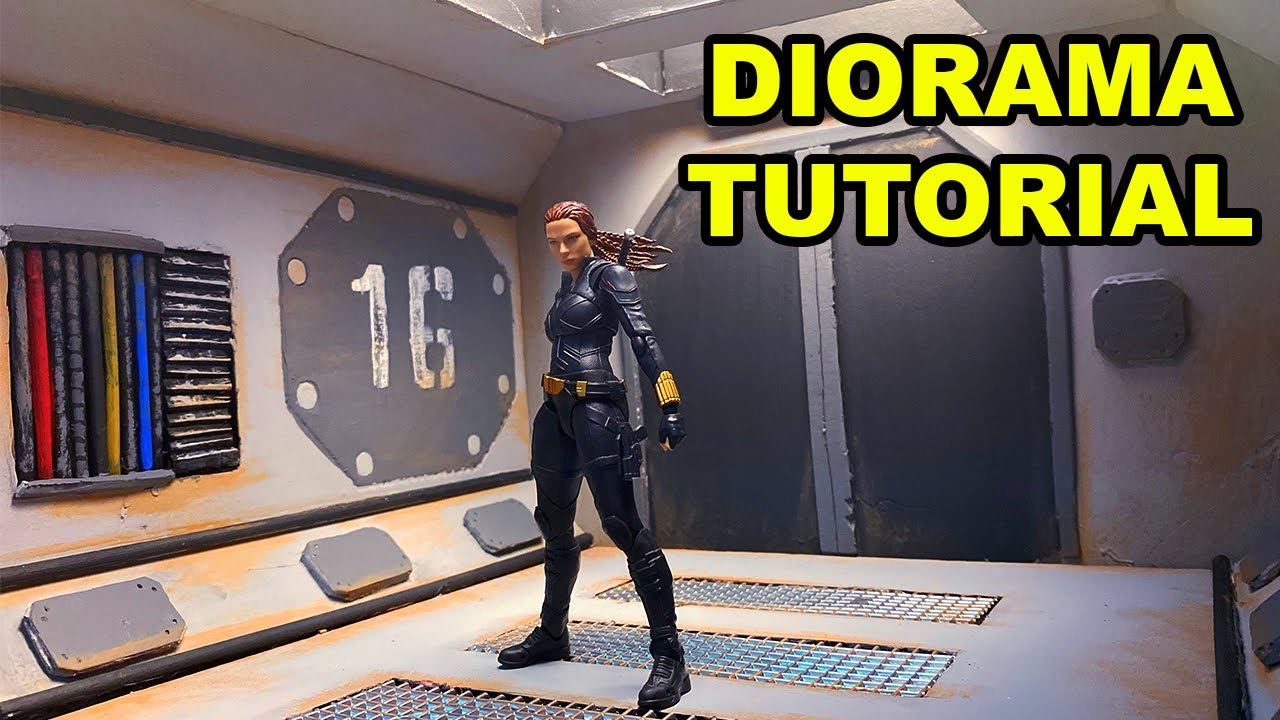The image portrays a still from a video game featuring a female character reminiscent of Tomb Raider inside a spaceship corridor. The corridor has silver-gray walls with darker gray outlines and two prominent black doors. A gray metal plate with the number "16" in white is affixed to the left wall, alongside a window adorned with colorful fabric lines in red, blue, and gray. On the bottom of the wall are metallic oblong objects. The character is centrally positioned, wearing a full black leather outfit, including high knee boots, a red belt buckle, and gold wristbands. She has a brown ponytail that appears to blow to the side despite no visible wind source. Her left arm is visible with a pistol on her left hip, while her right arm is obscured. A sword handle with a round silver tip and black grip is noticeable between her back and hair. The floor beneath her is tan with three silver grates. At the top of the image, yellow bubble text reads "diorama tutorial."